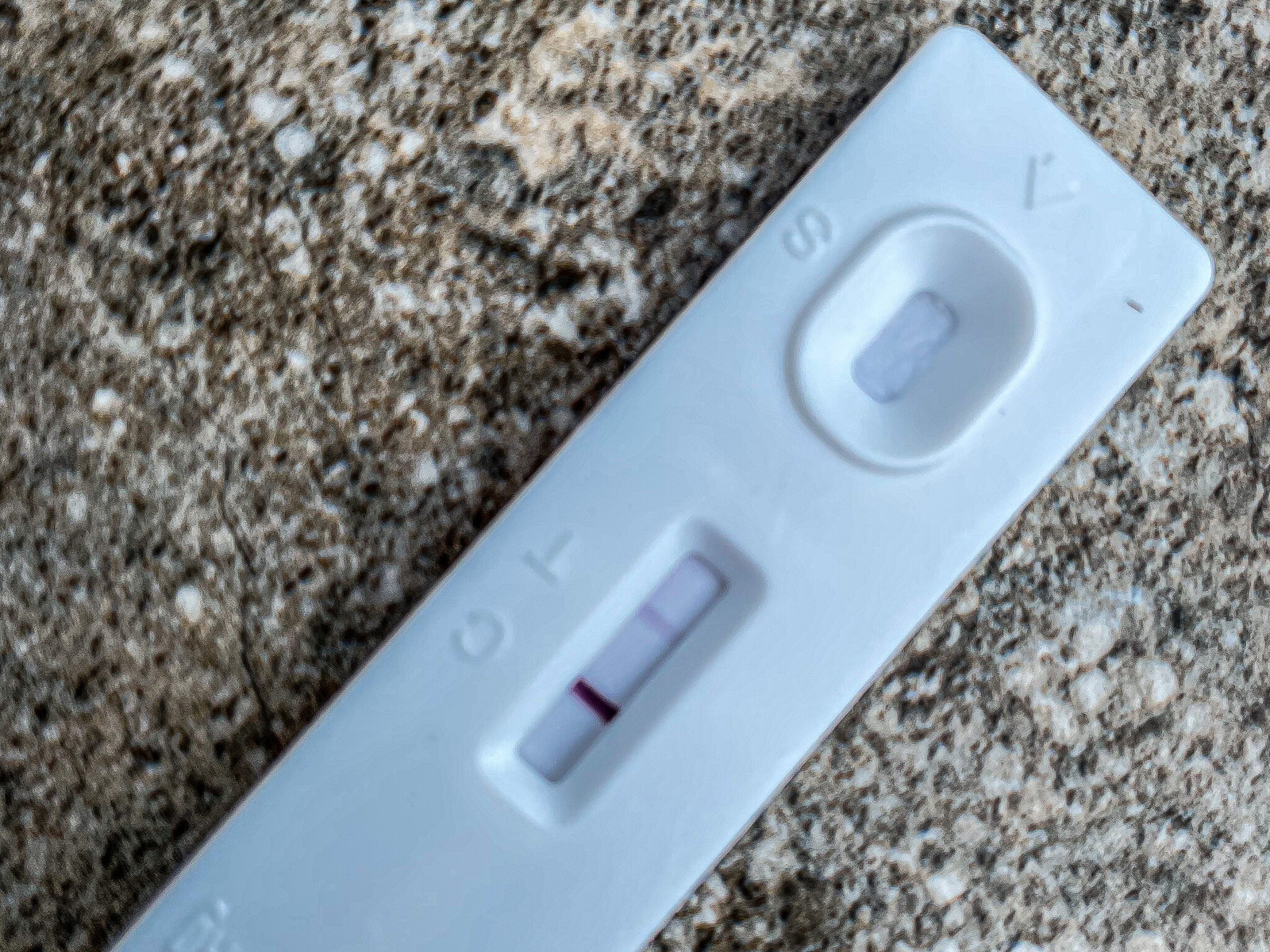In this close-up image, a home pregnancy test is positioned diagonally on a marble-like counter. The countertop features a speckled pattern of brown, white, cream, and a hint of black, resembling a natural stone surface. The pregnancy test itself shows a positive result. It has two windows labeled with letters C, T, and S. The window labeled with C (likely indicating "control") displays a dark red line, while the window with T (likely indicating "test") shows a lighter pink line, confirming a positive result. The third window with the S label appears empty, marked only by an oval shape with a rounded rectangular outline and an arrow pointing towards it.